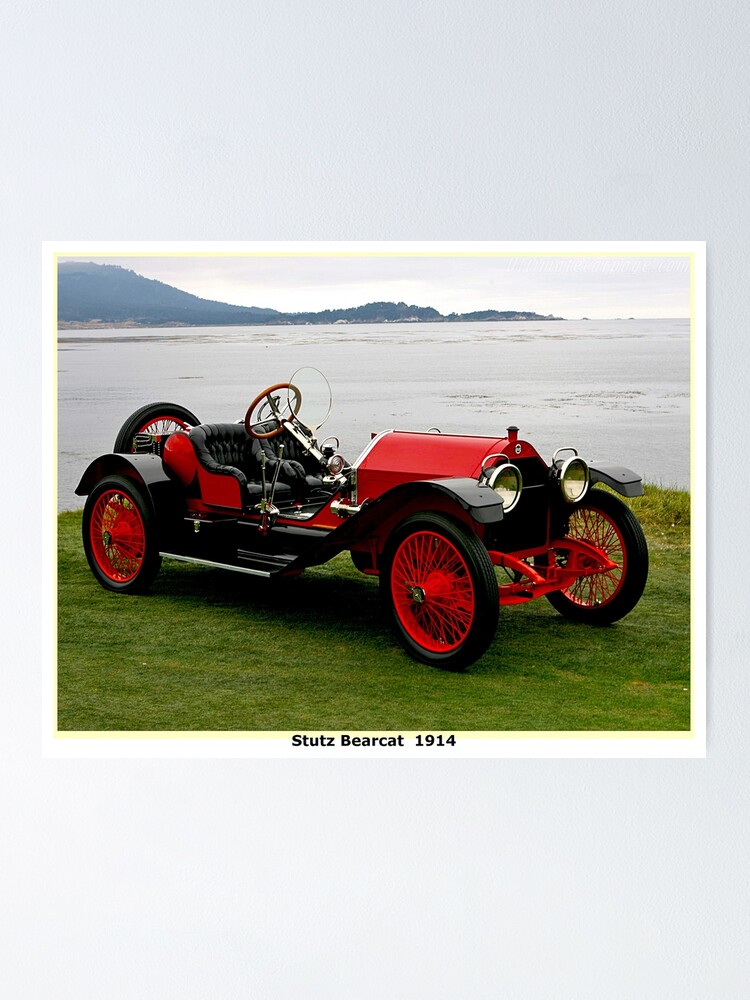This image captures a beautifully preserved 1914 Stutz Bearcat, an iconic early automobile. The vehicle, with its striking red body, black fenders, and chrome detailing, is showcased without doors or a roof, typical of its vintage open-roadster style. Notable features include a large brown steering wheel mounted on a chrome column and luxurious black leather interior. The car's red hood is complemented by two prominent chrome circular headlights and black tires accented with red rims. Adding to the vintage charm, a spare tire is mounted at the back of the car.

The Stutz Bearcat is set on a vibrant green grassy surface, with a serene grayish body of water and rolling mountains in shades of gray and purple in the background. These scenic elements are framed by a light gray sky, enhancing the timeless beauty of the photograph. The image is bordered by a white frame and placed on a light blue rectangle, giving it a postcard-like appearance. The entire composition focuses solely on the automobile and the picturesque natural setting, free from any other distractions or text.